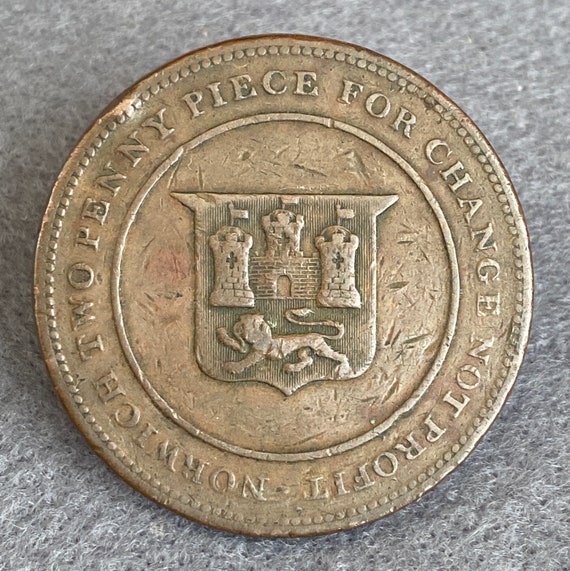This photo showcases a worn and old-looking bronze coin, closely resembling a penny, placed on a grey marble-like table. The coin features tiny circles lining its edges, followed by the inscription: "Two penny piece for change, not profit." Just inside this inscription, a single ring frames the central part of the coin, which is heavily scratched and dinged. In the center, a detailed crest depicts a castle with three towers, each adorned with a flag and cross-shaped windows, and beneath the castle stands a lion with its tail raised and paw extended. This entire crest is enclosed within the shape of a shield, reflecting the coin's historical and intricate design.